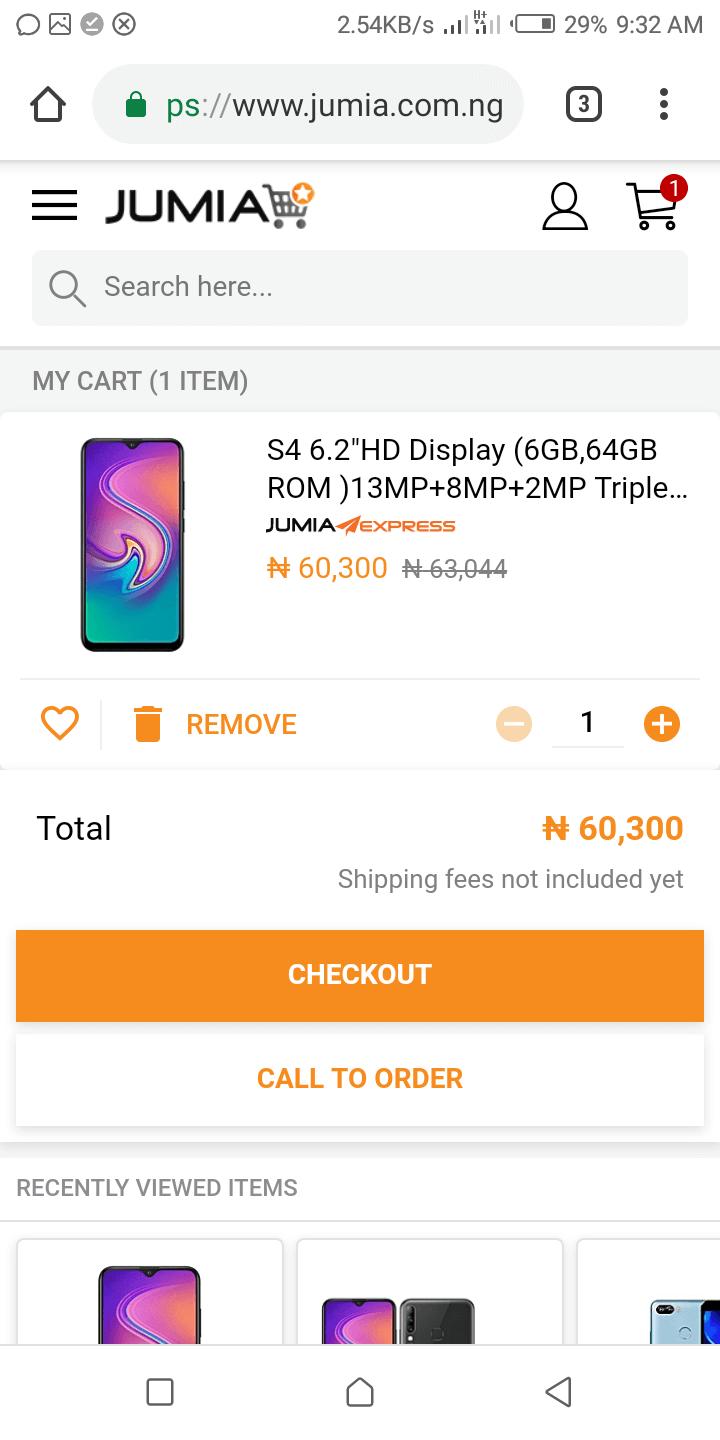This screenshot captures a smartphone display with a white background, including the top header. In the top header, the time displayed on the right side reads 9:32 AM. Adjacent to the time is the battery icon indicating a 29% charge, followed by two wireless connection icons. The data transfer rate is shown as 2.54 KBS next to these icons.

Below the top header, the web address in focus is "jumia.com.ng." Directly beneath this is the Jumia logo, clearly signifying that the screenshot is from Jumia's e-commerce site. The Jumia logo features the company name "JUMIA" in bold, black capital letters, accompanied by a small black drawing of a shopping cart, representing the company's identity.

On the right side of the header, there are two icons: an account icon and a shopping cart icon. The shopping cart icon has a red circle with the number "1" inside it, indicating that there is one item in the shopping cart.

The central content of the screenshot displays the details of the item in the shopping cart. On the left side, there is an image of a smartphone with an abstract swirling design on its screen, blending blue at the bottom with purple and orange at the top. The smartphone is labeled "S4 6.2 HD display," and additional specifications listed include "6 KB" and "64 GB ROM," among other details.

Towards the bottom of the screen, an orange rectangular button is prominent, featuring the text "Check out" in white, inviting the user to proceed with their purchase.